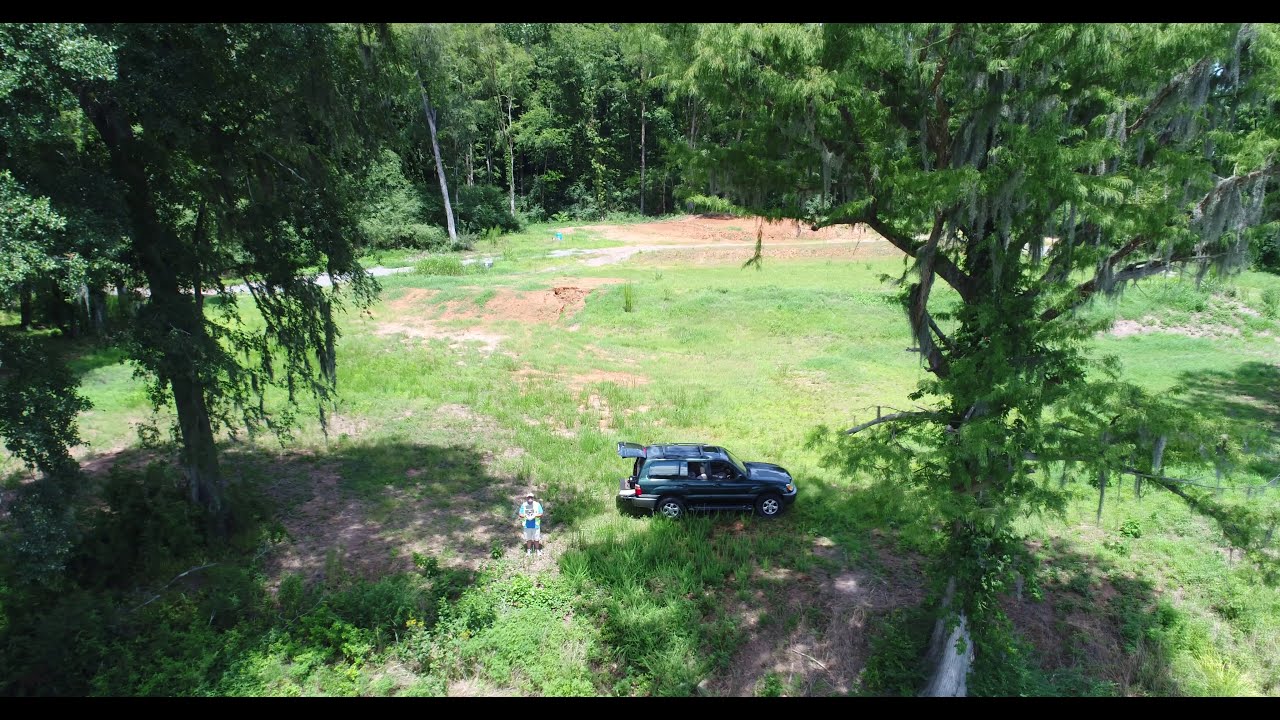The image captures an aerial view, likely taken from a drone, showcasing a secluded clearing in the midst of a dense forest. The sunlight illuminates the area, highlighting a mix of lush green grass and patches of reddish-brown soil devoid of vegetation. In the center of this clearing stands a man, identifiable by his white hat, light blue shirt, white pants, and white shoes. He is gazing directly at the camera, approximately 20 to 30 feet away. Nearby, there is a green Land Rover-type SUV with its back door open, revealing its silver and thick rims. The high grass and weeds that surround the clearing are bordered by rows of tall trees, adding depth to the forested backdrop. The man appears to be holding a controller, suggesting he might be operating the drone capturing this detailed and serene moment in the woods.